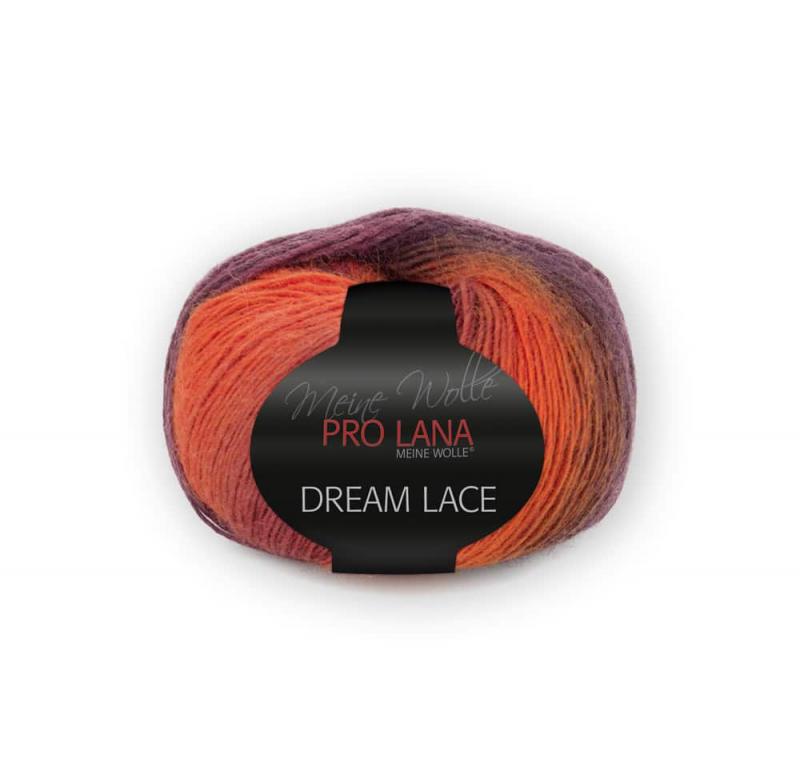This image features a centered ball of yarn set against a solid white background. The yarn, primarily amber-colored with hints of orange, transitions into shades of brown and flecks of red and purple. The yarn is packaged with a prominent black label, vertically spanning from top to bottom. The label includes several inscriptions: at the top, in elegant cursive gray letters, it reads "Meine Wolle." Below that, in bold, all-caps red letters, it states "Pro Lana." Underneath "Pro Lana," in small white print, the words "Meine Wolle" appear again. Finally, at the bottom of the label, in large white capital letters, it declares "Dream Lace." The yarn has a translucent, slightly shiny texture with visible circular lines radiating around the label, giving it a distinct and layered appearance.